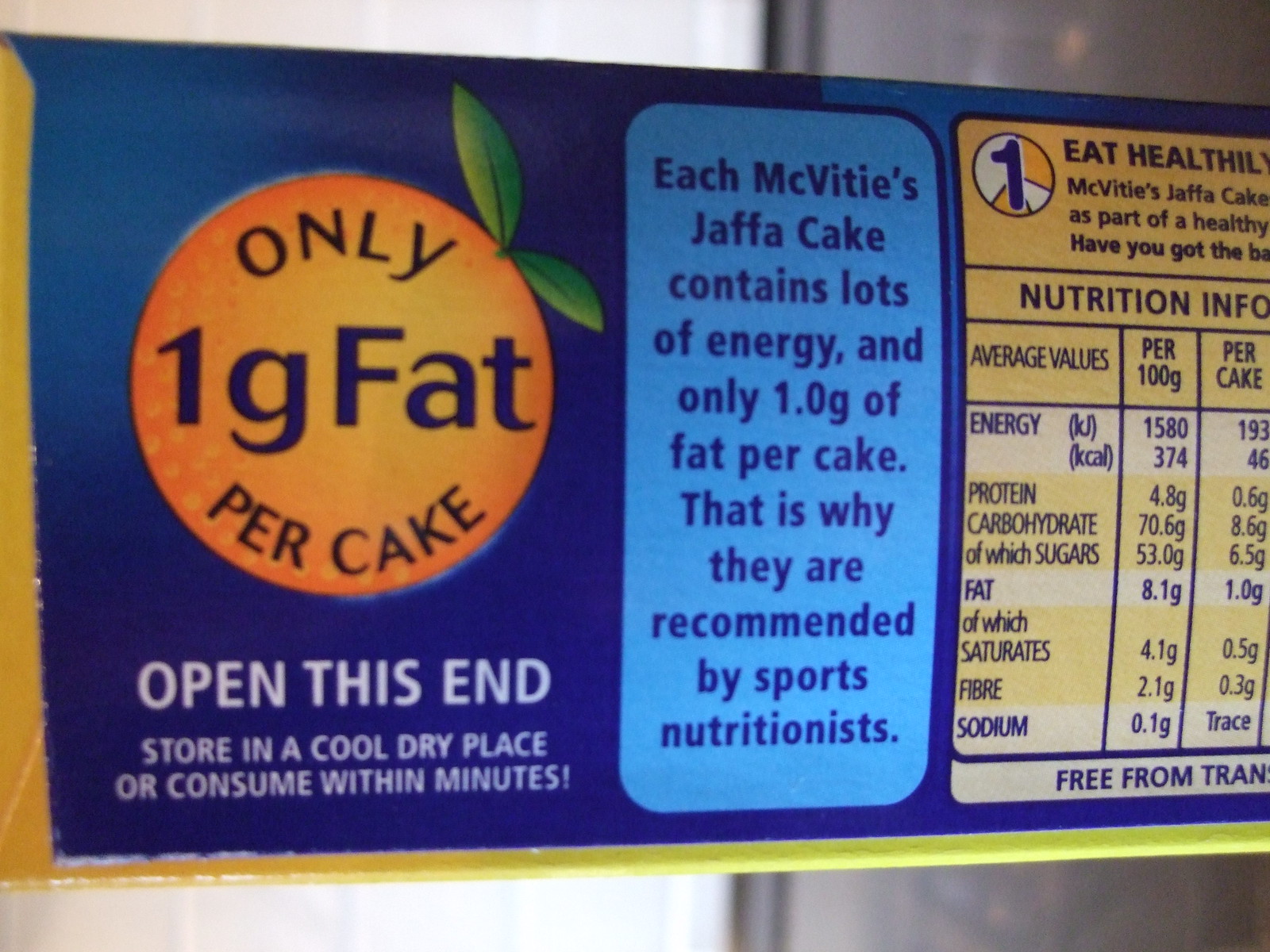The image is a close-up of the back label of a McVitie's Jaffa Cakes package, captured in a horizontal rectangular photograph. The background of the scene is divided, with a white wall on the left side and a grayish dark wall on the right. The product label, occupying about 90% of the image's center, features a predominantly blue background with distinct sections for different information.

On the left side of the label, there's a bright orange circle with two green leaves on its top right, representing an orange fruit. Inside the circle, text in dark blue or black font states, "only 1g fat per cake." Below the orange circle, additional instructions in white text on a blue background read, "open this end, store in a cool dry place or consume within minutes."

To the right of this section, a vertical light blue rectangle contains the product's promotional message in dark blue text: "Each McVitie's Jaffa Cake contains lots of energy and only 1.0g of fat per cake. That is why they are recommended by sports nutritionists."

Finally, on the far right, there is a vertical yellow panel filled with nutritional information written in blue text, arranged in five or six lines. Overall, the label blends vibrant colors and clear text to convey essential product details and make the packaging visually appealing.